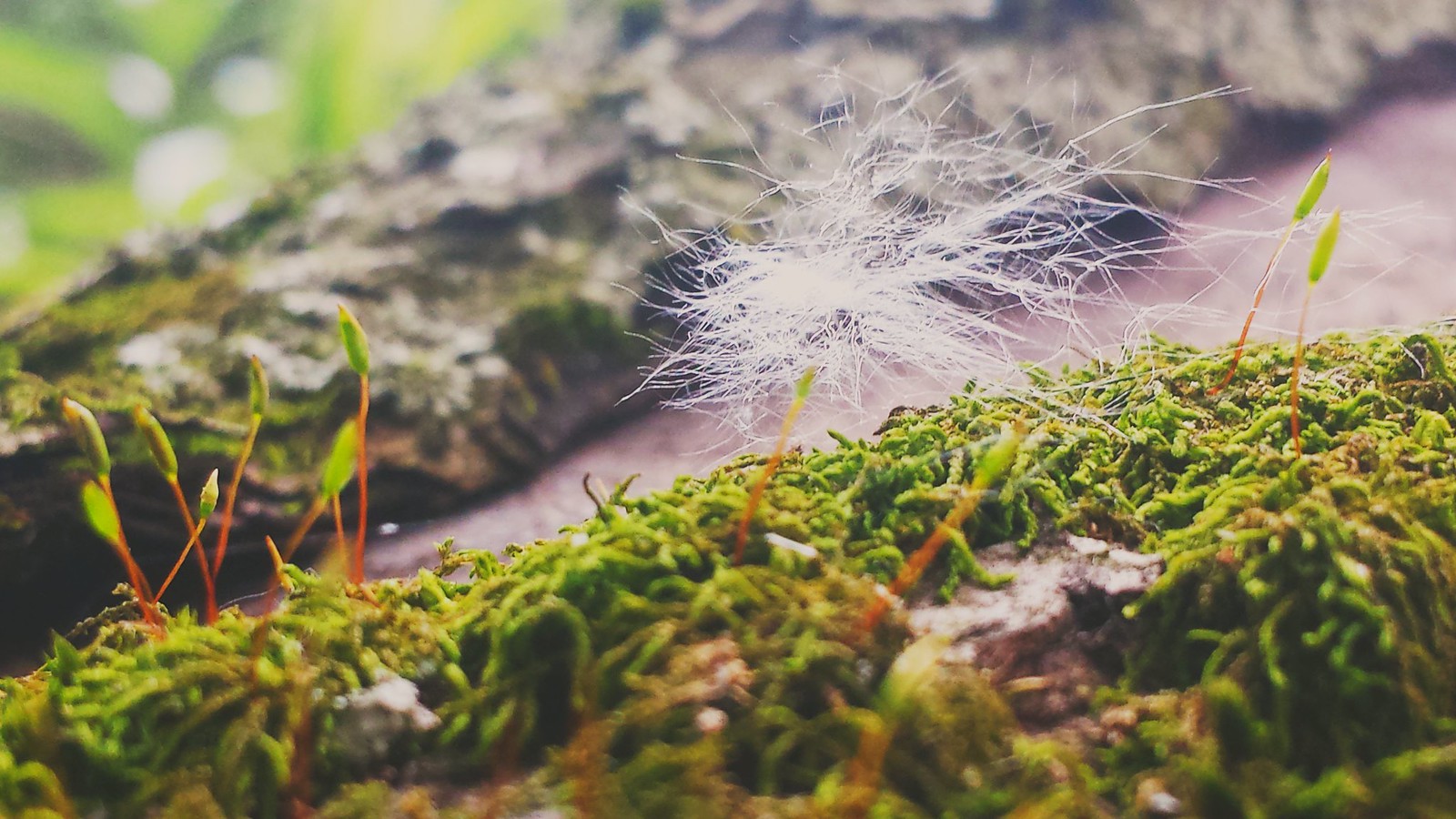The close-up photograph reveals a detailed view of a forest floor covered in vibrant green moss. The perspective highlights the intricate texture of the moss, appearing as tiny green strings densely packed together, extending from the lower left to the middle right of the image. Emerging from the moss are several delicate brown stems, each crowned with small green bulbs, resembling tiny sprouts. Dominating the center of the image is a conspicuous clump of airy, white filaments, similar to dandelion fuzz or animal hair, adding a contrasting texture to the scene. In the background, a wet gray rock or possibly tree bark lies horizontally, its rough surface accentuating the lush vegetation in the foreground. The upper left corner of the image is blurred, showcasing bright green leaves that add a splash of color to the scene. The photograph, a horizontal rectangle, captures the minute details of the forest floor with an intimate and almost surreal closeness.